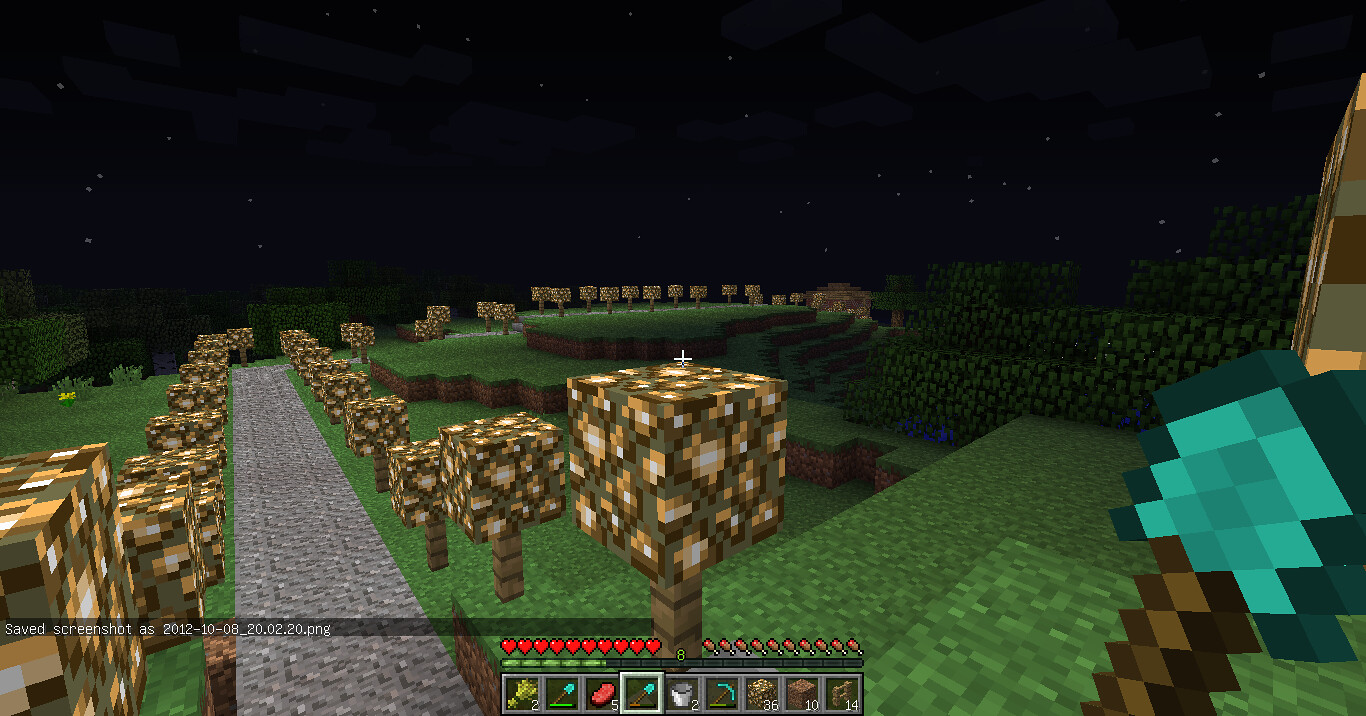The image is a color screenshot from the game Minecraft capturing a wide, panoramic landscape. An overlay of text appears slightly above the bottom left corner on a translucent dark grey background, with white font that reads "2012-10-08" followed by "20.20.png" with a slight space between them. The central part of the screenshot displays various inventory icons: a bundled branches icon, a spade icon, a bucket icon marked with the number 2, and a pickaxe icon with a brown handle and green head. The top left corner of the image features a series of heart icons, while the top right shows chicken leg icons, representing health and hunger levels, respectively.

The in-game landscape depicted in the screenshot consists of multiple layers, starting with a grassy terrain. Square-shaped trees or bushes line a path that winds into the distance on the left side of the image, creating a sense of depth and exploration. The scene is quintessentially Minecraft, with its blocky, pixelated aesthetic and vibrant colors.